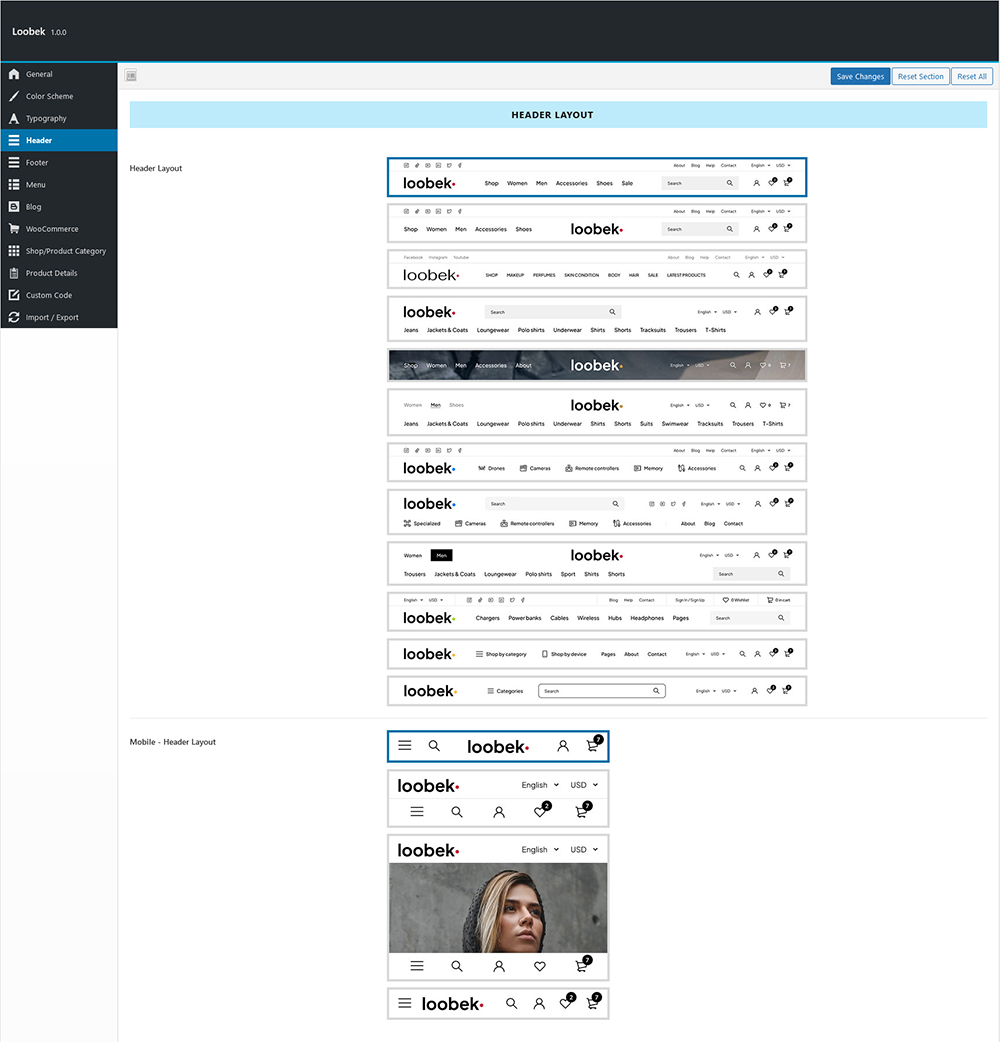Screenshot of the photo editing website, Lubec 1.1, displaying a user interface designed for creating posters with integrated image and text editing tools. The website provides various prompts for customization, such as options for larger and smaller font sizes and more stylized font choices. The user is currently typing a header and is shown several mobile header layout options, some of which have been previously favorited. The interface also includes a section for uploading an image, where the user has selected a picture of a woman with blonde hair wearing a grey hoodie. This image may be relevant to the intended header title.